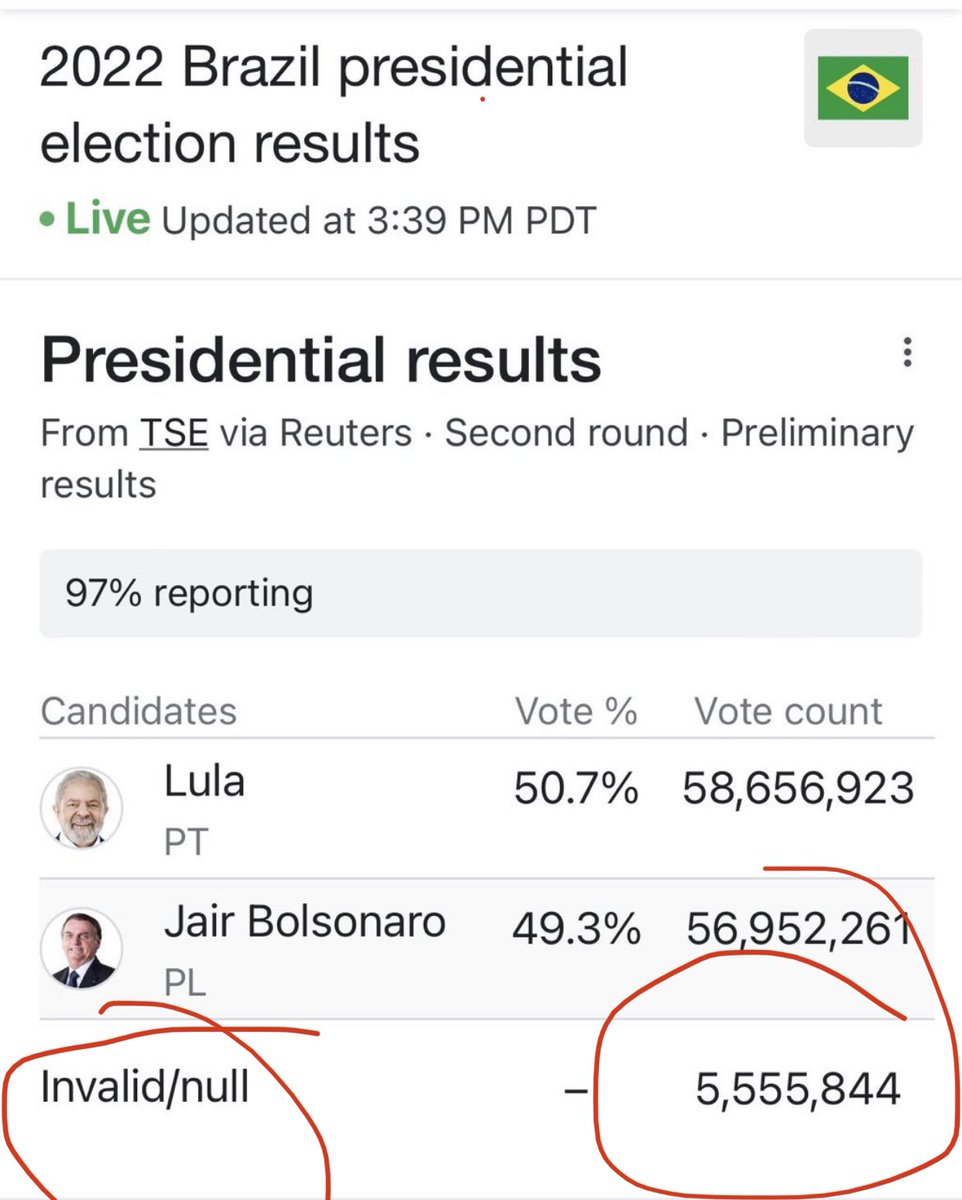This image captures a mobile display of the 2022 Brazil presidential election results. At the very top, the title reads "2022 Brazil Presidential Election Results," followed by a timestamp indicating the data was last updated live at 3:39 PM PDT. A Brazilian flag adorns the top-right corner, and the word "LIVE" is prominently highlighted in green, accompanied by a small green dot signaling real-time updates.

Just beneath the header, the webpage attributes the "Presidential Results from TSE via Reuters, Second Round Preliminary Results." The reporting progress is marked at 97%. 

The webpage details the results of the two main candidates:
- **Lula (PT)**: Lula holds a slight lead with 50.7% of the vote, totaling 58,656,923 votes.
- **Jair Bolsonaro (PL)**: Jair follows closely with 49.3% of the vote, amassing 56,952,261 votes.

Additionally, the page includes a section for invalid or null votes, quantified at -5,555,844.

The image itself seems to be captured from a mobile device, providing a clear and comprehensive overview of the election results as they stand at the specified update time.